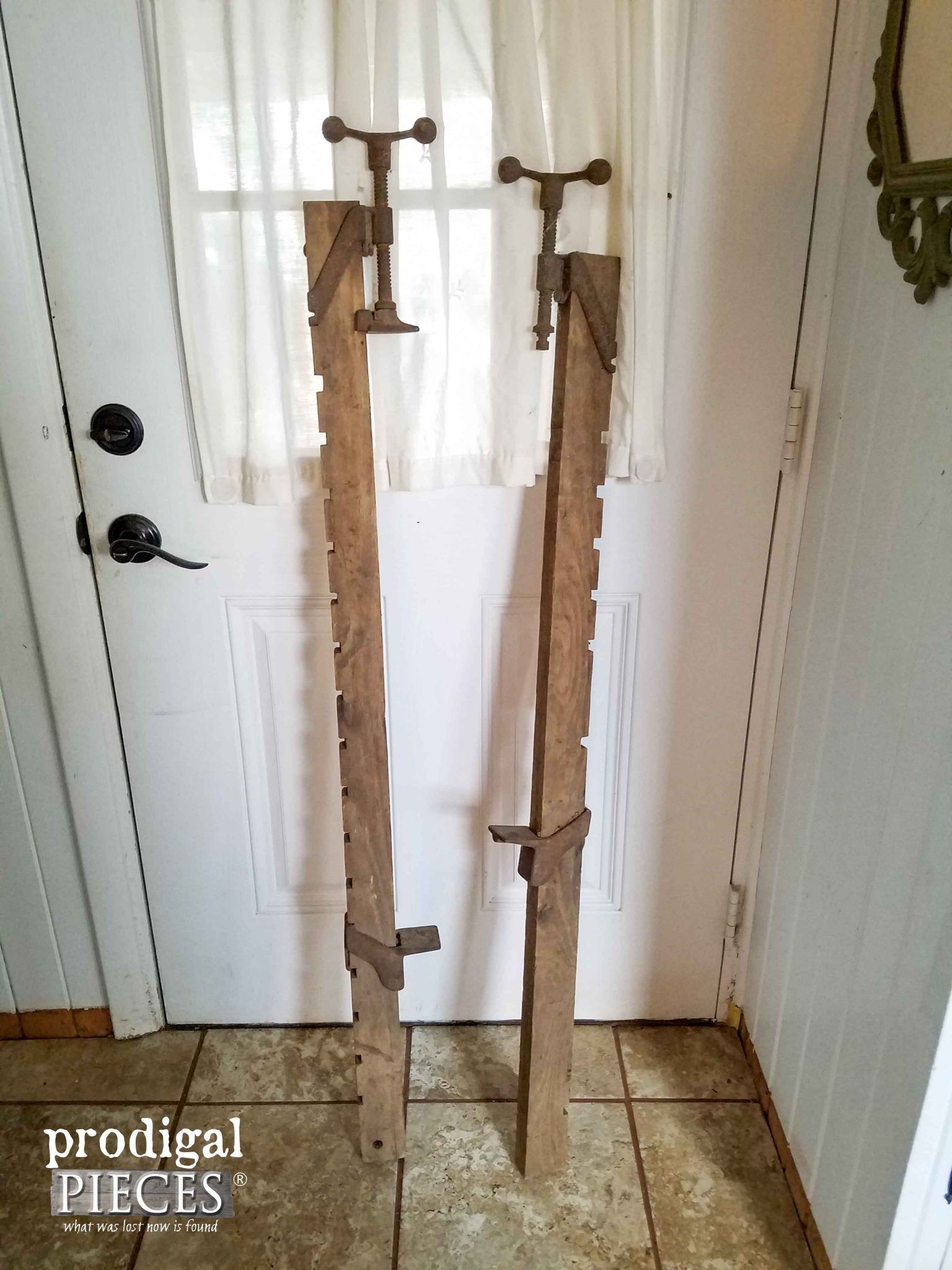The photograph features a white door with a black handle and lock, adorned with a window draped in white curtains. The surrounding trim and the door itself appear to be quite dirty. Leaning against this door are two identical long brown wooden objects with intricate notches along their sides and metal components fitted into these notches. Each of these wooden pieces has a metal piece with a turning contraption on top, suggesting they might be old clamps. The door is situated against a white wood wall and stands on a brown tile floor. To the right of the door, an antiquated, ornate mirror partially comes into view. In the bottom left corner of the image, there's text that reads, "Prodigal Pieces: What was lost now is found," adding a hint of mystery and nostalgia to the scene.